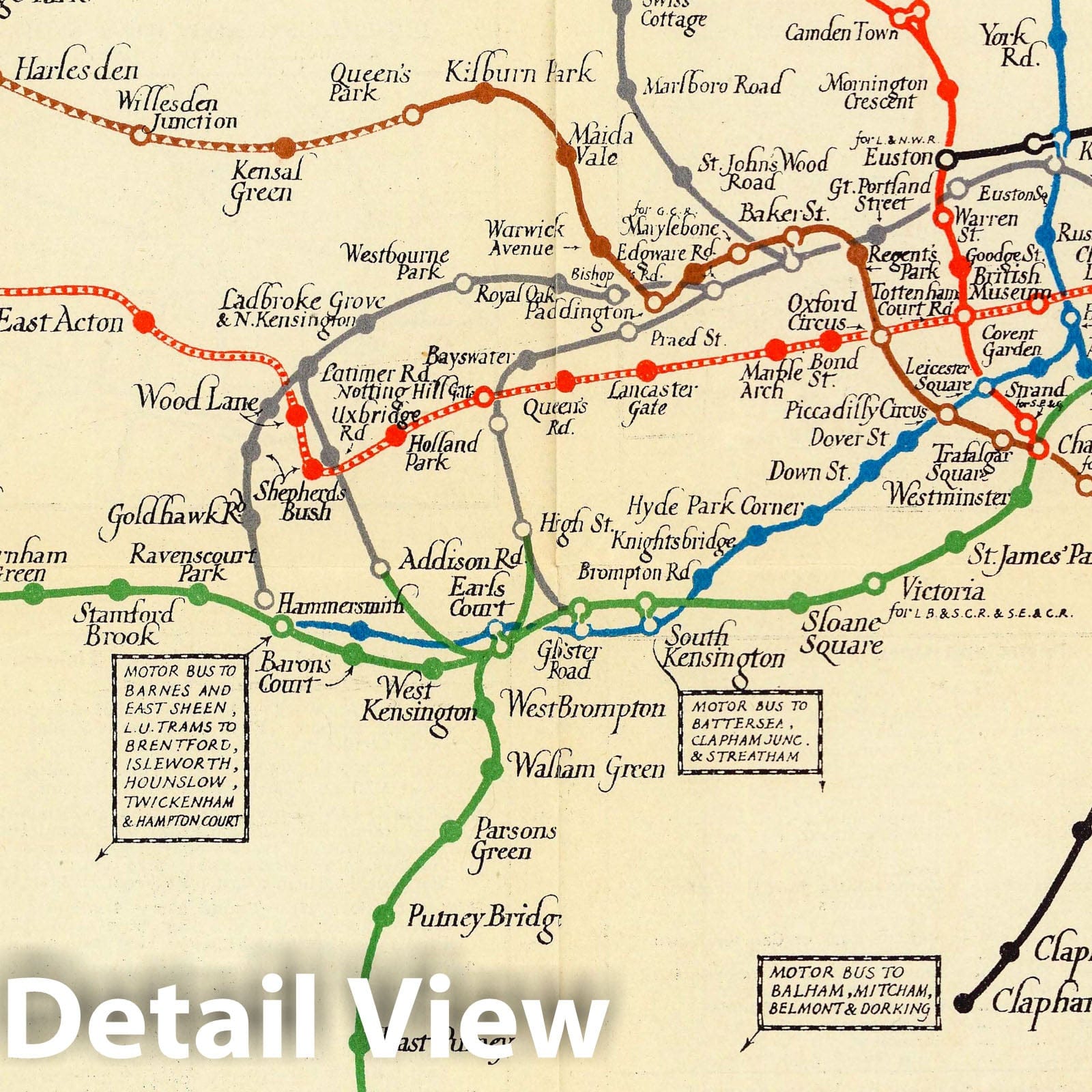This image depicts an old, detailed map set against an off-white, cream-colored background. Displayed prominently in large white font at the bottom left, the map is labeled "Detailed View." The map is intricately marked with various routes represented by squiggly lines in multiple colors—brown, red, gray, blue, and green—indicating different transportation paths, possibly for a train or subway system. Smaller black text labels various towns and destinations, although the writing is somewhat difficult to read due to its size. Notable locations include Kilburn Park at the top center and Earl's Court centrally located, along with other areas like Gold Hawk, Ravens Court Park, Hammersmith, Addison Road, and Hyde Park Corner. Additionally, the bottom section features a rectangle with text indicating "Motor Bus to Balham, Mitcham, Belmont, and Dorking," along with various other specified routes like to Barnes and East Sheen, and to Battersea, Clapham, Young, and Streetham. The map conveys an intricate network of destinations, hinting at an old, comprehensive transportation system.